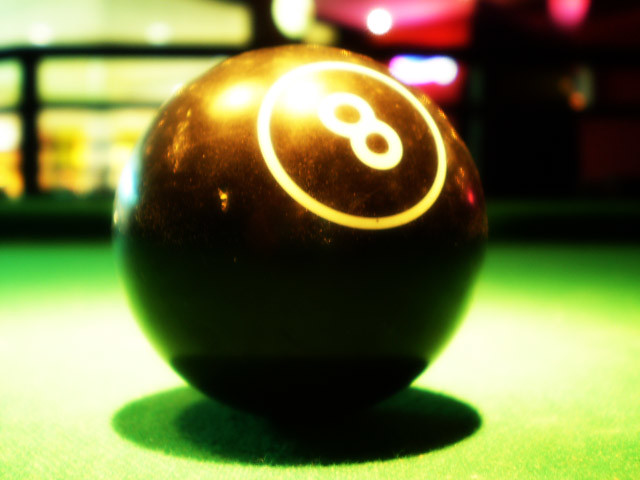This detailed color photograph captures a close-up of a black 8-ball from a pool table. The black 8-ball, prominently displayed in the center of the image, features a white ring and a white number 8 inside the ring. It rests on the green felt surface of a billiards table, directly under an overhead light that casts a distinct circular shadow beneath the ball. The surrounding background is blurred, but you can discern a shop setting that could be a bowling alley, pub, or pool bar, with out-of-focus elements such as windows, red and light green signs, and possibly other lights in yellow and black hues. Reflections from the overhead light create a gleaming effect on the 8-ball, emphasizing its polished surface. The ball is oriented such that the white circled 8 points toward the top right corner of the frame.